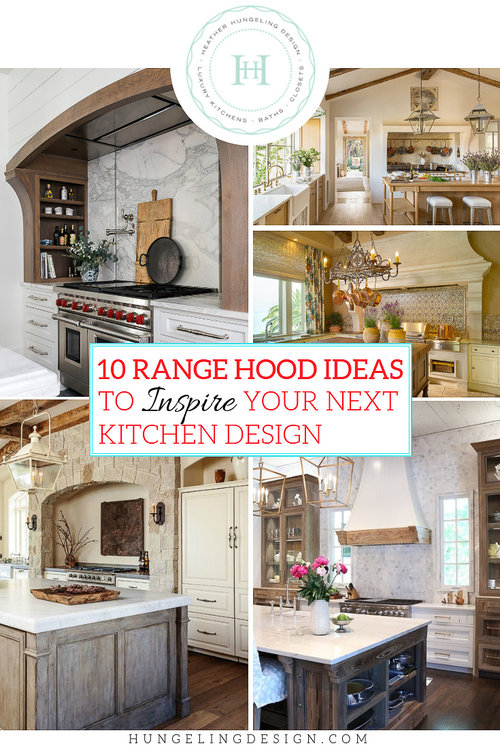The photo collage features a series of five beautifully designed kitchen images arranged in a grid pattern. At the top of the collage is a circular, white logo with an "H" symbol, labeled "Hever Hungling Design, Luxury Kitchens, Baths, and Closets." Centrally located within the collage is a white text box stating, "10 range hood ideas to inspire your next kitchen design." Each featured kitchen showcases elegant cabinets, refined lighting, and various kitchen utensils, reflecting luxurious and diverse design styles. Notably, one kitchen includes a stove set within an alcove, while another exhibits a more conventional layout. Across all images, the sophistication and high-end nature of the designs are evident.